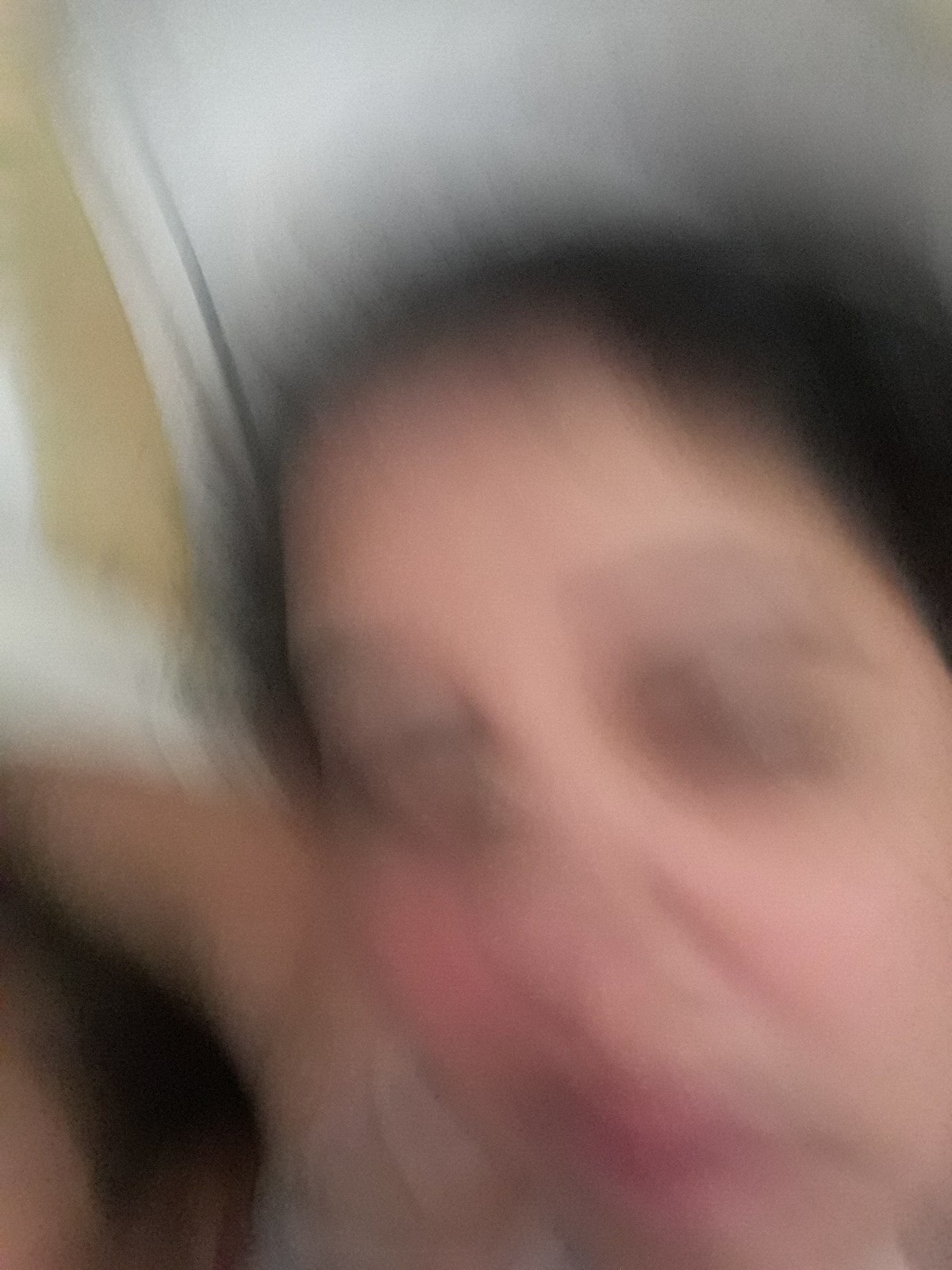The photograph depicts a person with dark hair, though the image is extremely blurry. The individual's face is partially visible, with their forehead, eyebrows, and nose discernible amidst the indistinct features, while their chin and the left side of their cheek are cut off by the edges of the photo. The eyes are shrouded in shadows, making it difficult to determine if they are open or closed, although the absence of visible whites suggests they might be closed. The pink hue of the mouth is faintly visible, but its exact contours are indeterminable. The person appears to have an arm extended either behind them or resting on the back of a chair or couch. Overall, the photograph's poor quality renders many details indistinct and obscured.